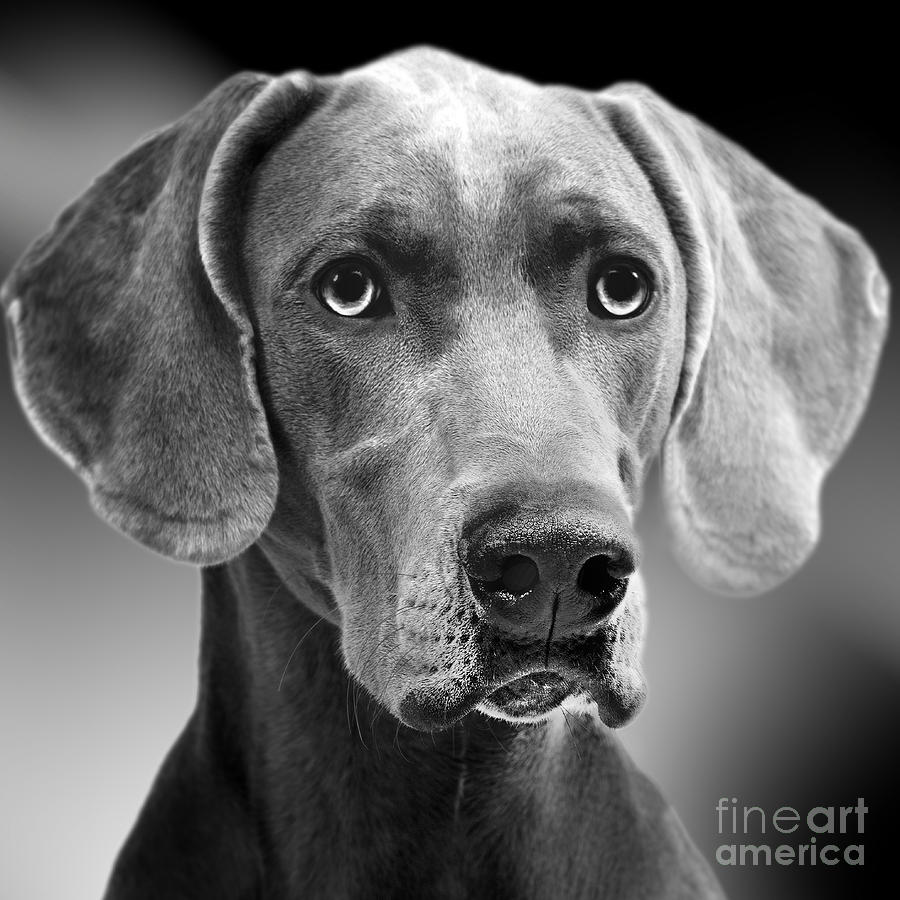This professional black and white photograph captures a close-up of a Weimaraner dog's face in exquisite detail. The dog, with its characteristic angular features and floppy ears, extends its dark-furred neck and shoulders to the bottom of the frame. The shades of gray meticulously exhibit the texture of its fine fur, accentuating a long snout and a pronounced black nose. Its round, soulful eyes and arched eyebrows impart a poignant, almost sad expression. The dog gazes slightly to the right of the viewer while the background remains blurred, highlighting the subject's contemplative pose. A subtle stamp in dark white letters at the bottom right corner reads "Fine Art America."